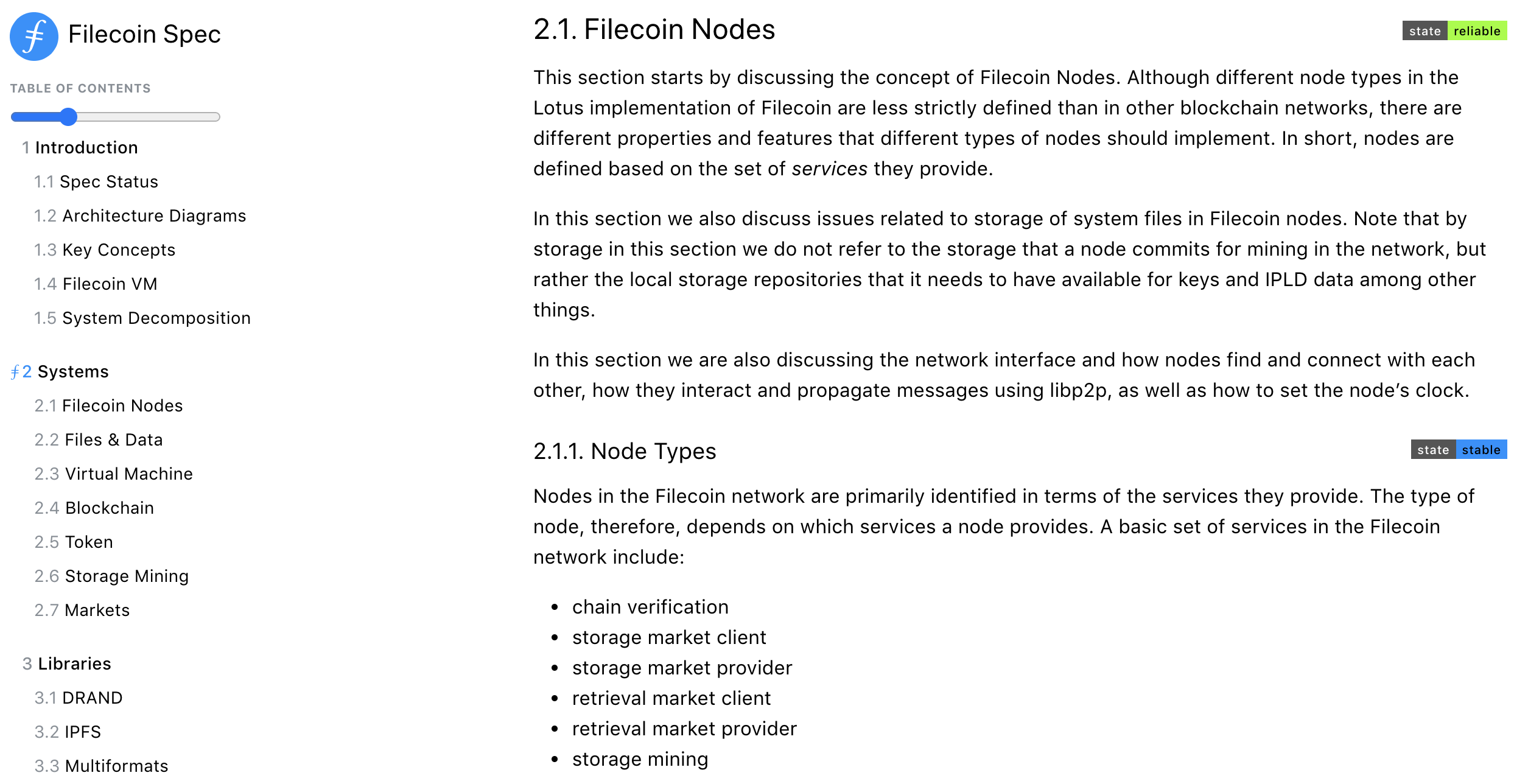In the upper left-hand corner of the image, there is a detailed screenshot titled "Filecoin Specification." Below this title, a structured table of contents is presented. The table of contents is prominently displayed within a rectangular box featuring a blue progress bar that fills approximately one-quarter of the box from the left. The contents are divided into three comprehensive sections:

1. **Introduction**: Spanning from subsections 1.1 to 1.5, this includes various foundational elements such as "Spec Status," "Architecture," "Diagrams," "Key Concepts," "Filecoin VM," and "System Decomposition."
   
2. **Systems**: Covering subsections 2.1 to 2.7, this section elaborates on "Filecoin Nodes," "Files and Data," "Virtual Machine," "Blockchain," "Token," "Storage Mining," and "Markets." 

3. **More Systems**: This final section ranges from 3.1 to 3.3, addressing "Transport (TRN)," "InterPlanetary File System (IPFS)," and "Multi-Formats."

On the right side of the image, subsection 2.1 titled "Filecoin Nodes" is expanded, displaying three paragraphs of explanatory text. The content then transitions into subsection 2.1.1 labeled "Node Types," which includes one paragraph of descriptive text along with some bullet points. This fragmented view provides a glimpse into the detailed and organized structure of the Filecoin technical documentation.